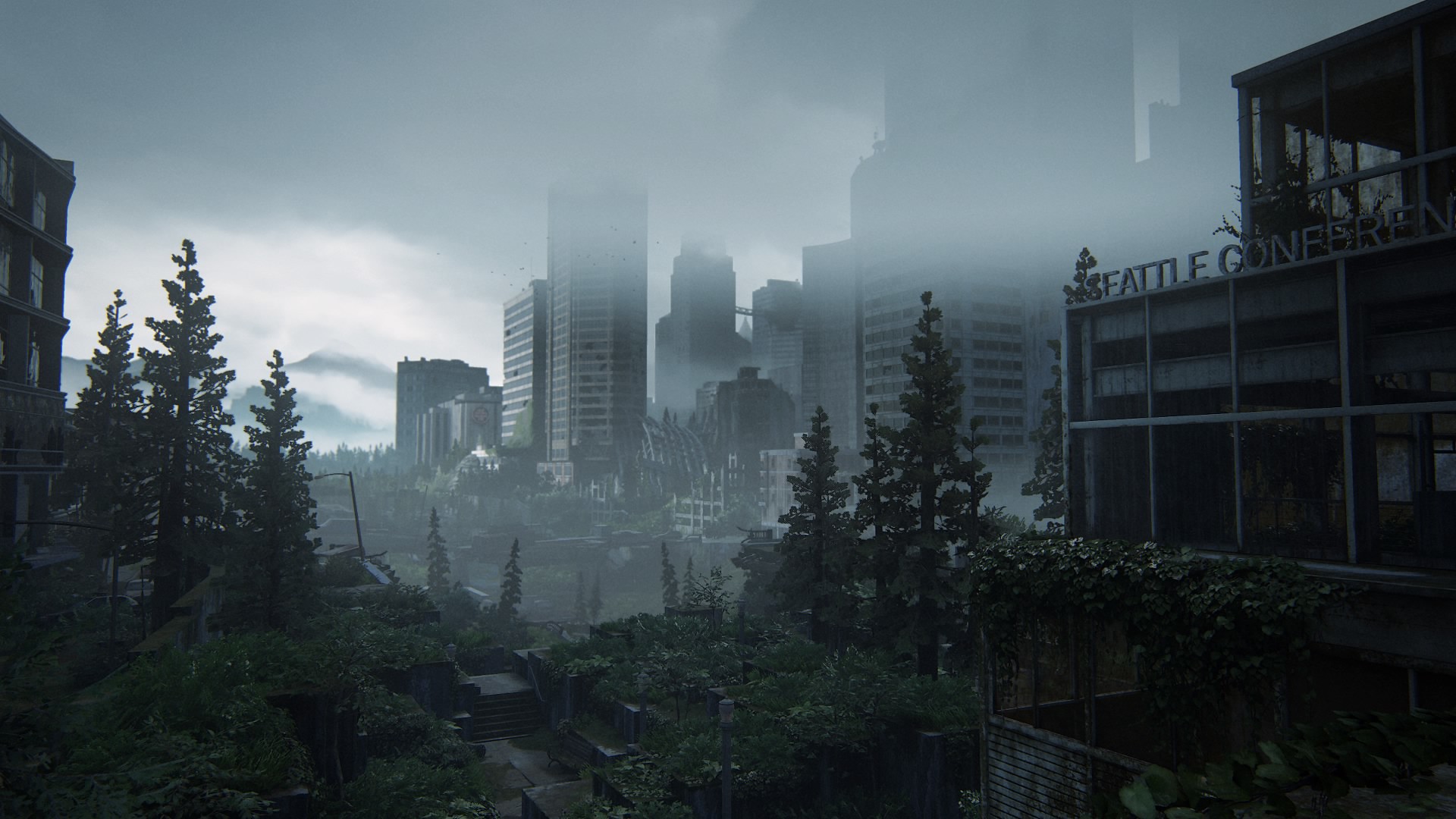In this image, a foggy cone barrier looms, shrouded in perpetual darkness with no hint of light breaking through. The sky above is a bleak, overcast gray, with distant clouds that add to the gloomy atmosphere. The urban landscape below is dotted with numerous high-rises, some with broken or missing windows, implying neglect and decay. One particular building appears to have collapsed from its foundation, caving in on itself completely. In the bottom left corner of the image, trees and overgrown vegetation are visible, showcasing how nature has started to reclaim the urban environment. Vines and plants can be seen creeping up and enveloping structures, including the Seattle Conference Center, which has an overgrown window, further emphasizing the theme of nature overpowering the city.